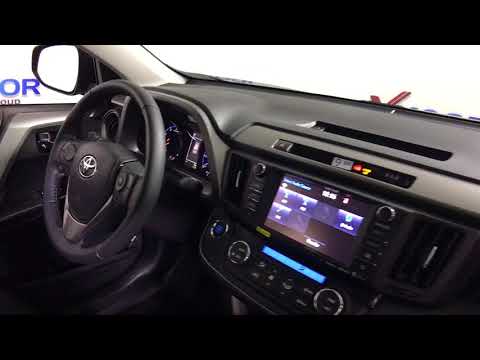The image depicts the interior of a Hyundai vehicle in detail, captured during the daytime. Central to the frame is a touchscreen display, likely functioning as a radio and showcasing various controls, which occupies a prominent position in the middle of the image. To the upper left is the steering wheel, accompanied by the driver’s side window and side mirror, partially visible alongside the rearview mirror. The windshield spans the top of the photo, further affirming the inside-the-car perspective. The dashboard area features knobs, possibly for temperature control, and a stick shift is also discernible. The color palette includes white, red, blue, gray, black, and silver hues, adding to the sleek and modern design of the vehicle's interior. Notably, there is blue labeling with “OR” in front of a white wall in the background, providing an unusual and intriguing detail. There is no visible text within the vehicle itself, suggesting the image might be part of a vehicle advertisement.